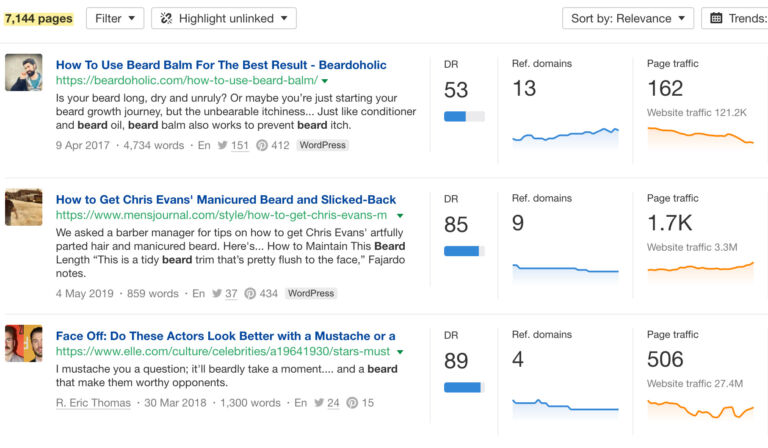The image showcases a webpage with a clean, white background, presenting a detailed list of website traffic statistics. In the top left corner, a highlighted box in light yellow indicates "7,144 pages." Adjacent to this, options labeled "Filter" and "Highlight Unlinked" are visible. Moving further right, there are additional options, including "Sort by Relevance," "Trends," followed by a light gray dividing line.

Below this header, the webpage lists different articles with associated metadata:

1. **"How to Use Beard Balm for the Best Results"** - Accompanied by an image of a bearded man. To the right, statistics on the domain and page traffic are presented.
2. **"How to Get Chris Evans' Manicured Beard and Slicked Back Hair"** - Displays page traffic of 1.7k and total website traffic of 3.3 million.
3. **"Face Off: Do These Actors Look Better with a Mustache or Without?"** - Shows page traffic of 506 and website traffic of 27.4 million.

Each entry provides a visual and numerical insight, aimed at evaluating the content's reach and popularity.